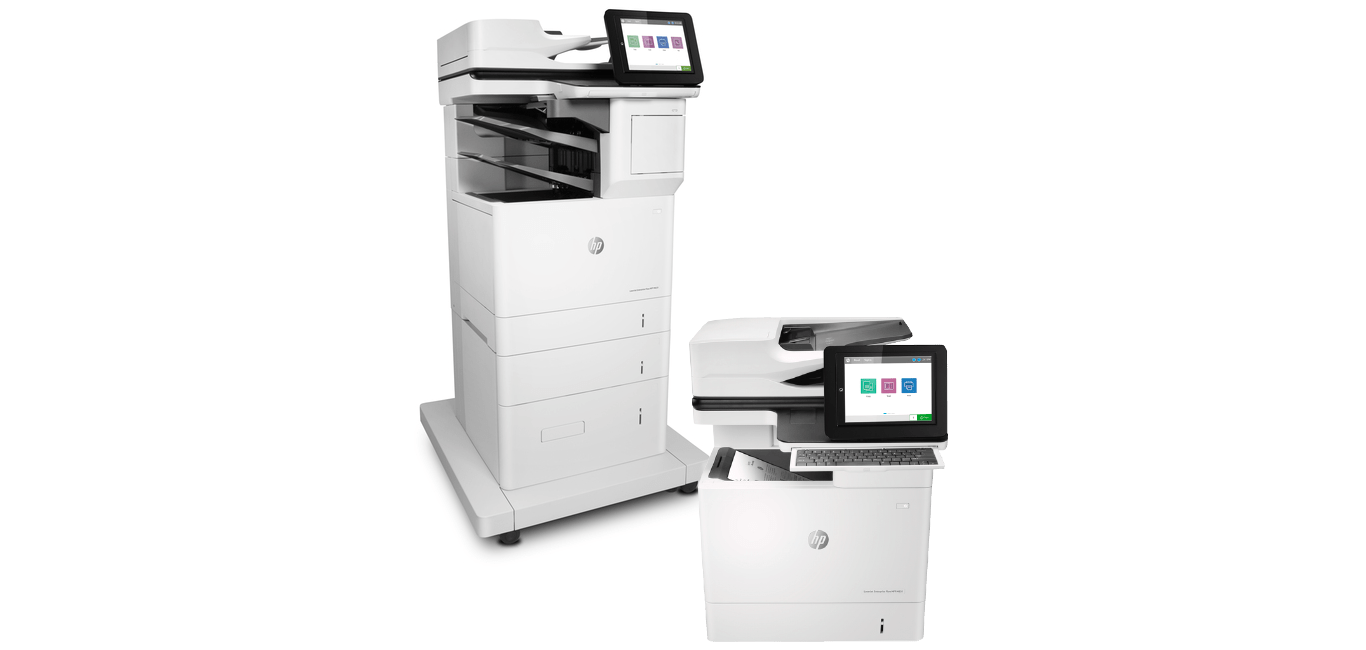In this image, we see two white HP office machines set against a white background, likely intended for advertisement. The larger machine on the left stands about waist-height and features a high-positioned copier unit with various slanted sorting racks below it, designed to manage and divide printed papers. This machine also includes a prominent digital screen at the top-right corner for user control, beneath which lies a large square component and three drawers, indicative of high-volume, professional printing capabilities.

Adjacent to it on the right is a smaller printer, approximately a couple of feet high, which appears to be a compact version or close-up of the top of the larger unit. This smaller printer is equipped with a similar top-mounted digital screen that displays vibrant teal, purple, and blue colors, hinting at its color printing and copying capabilities. Below the screen, there's a tray for printed paper and a square section likely for paper input. Both devices exude a high-quality finish typical of HP products, suggesting reliable and professional-grade performance.